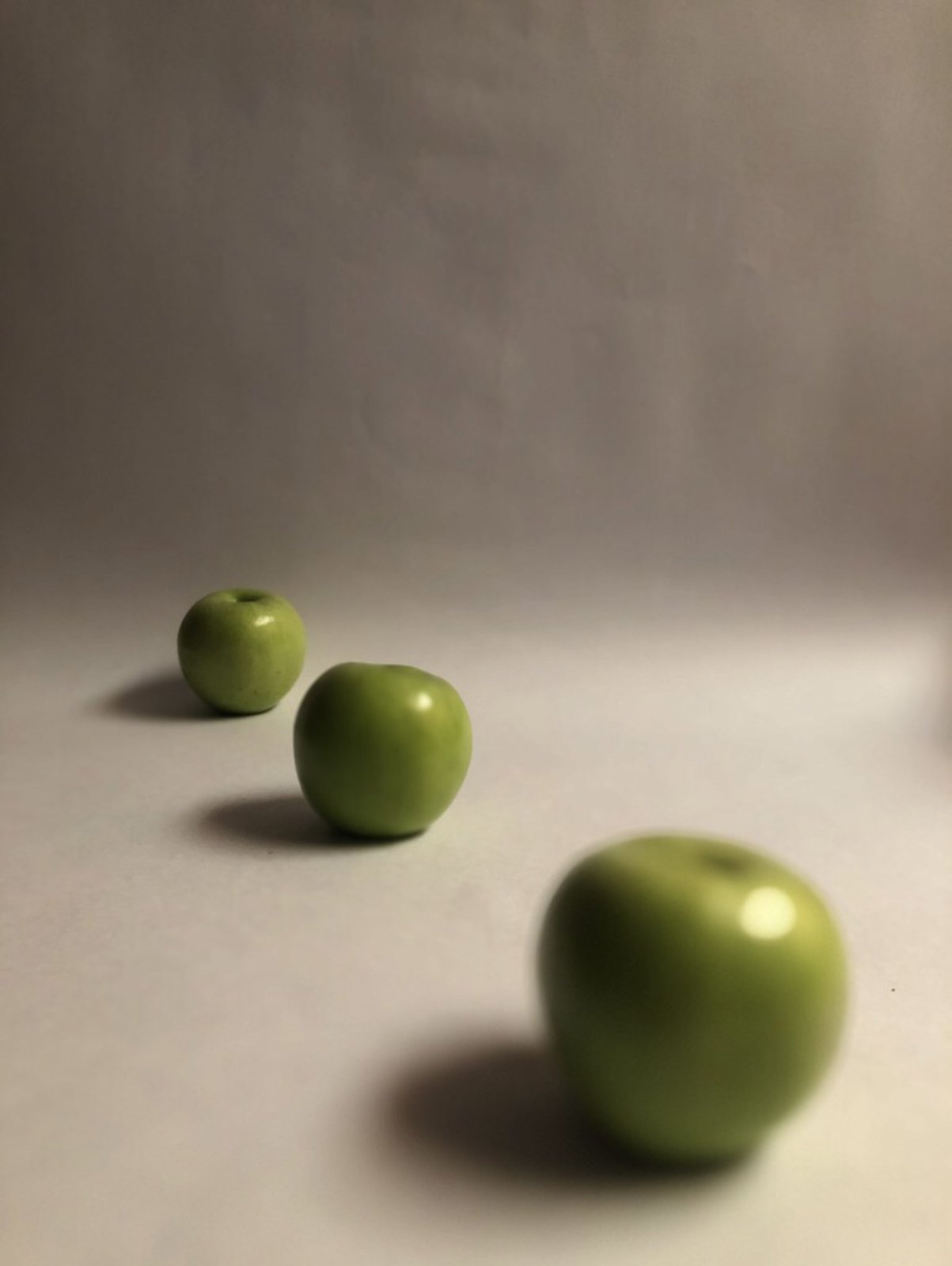In this image, three green apples—resembling Granny Smiths—are arranged in a row, each slightly spaced apart. The apples appear bright and shiny, with noticeable light reflections on their surfaces and distinct shadows extending behind them, suggesting a light source from the right. The first apple, positioned closest to the camera, is slightly out of focus but still appears intact and glossy. The middle apple is more in focus, offset slightly left of center, and exhibits a more prominent shadow. It has a round shape, though it shows a bit of unevenness. The third apple, set furthest from the camera, is the most visually prominent due to its perfect, round form and lighter green hue. All apples are displayed against a plain white backdrop that curves smoothly from a vertical to a horizontal plane, providing a clean and unblemished setting for the fruit. The ground where they are positioned appears brighter than the background, highlighting the apples' vibrant colors and textures.